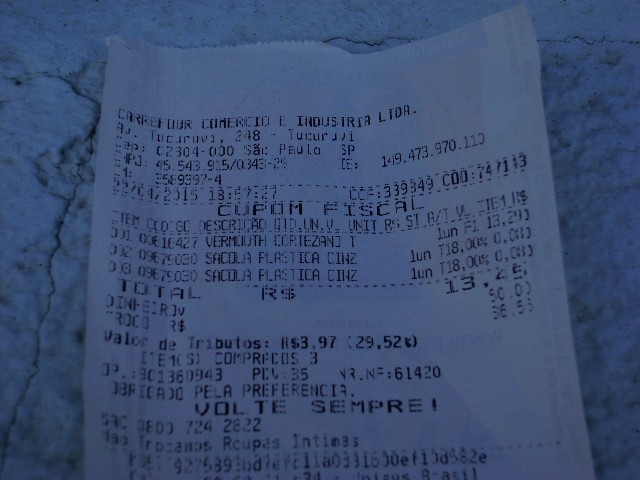The image captures the upper portion of a printed receipt laying on a cracked, grayish cement ground or possibly a marble countertop, both of which exhibit a bluish tint that suggests a filter was applied. The receipt, slightly rectangular and horizontally oriented, features black text, though some parts appear faded as if the printer was running out of ink. The details of the receipt are somewhat difficult to read, but visible text includes "Industrial TDA," "CUPOM FISCAL," and "VOLTE SEMPRE." The total amount listed on the receipt is $13.45. The majority of the text is in a language that appears to be Spanish.